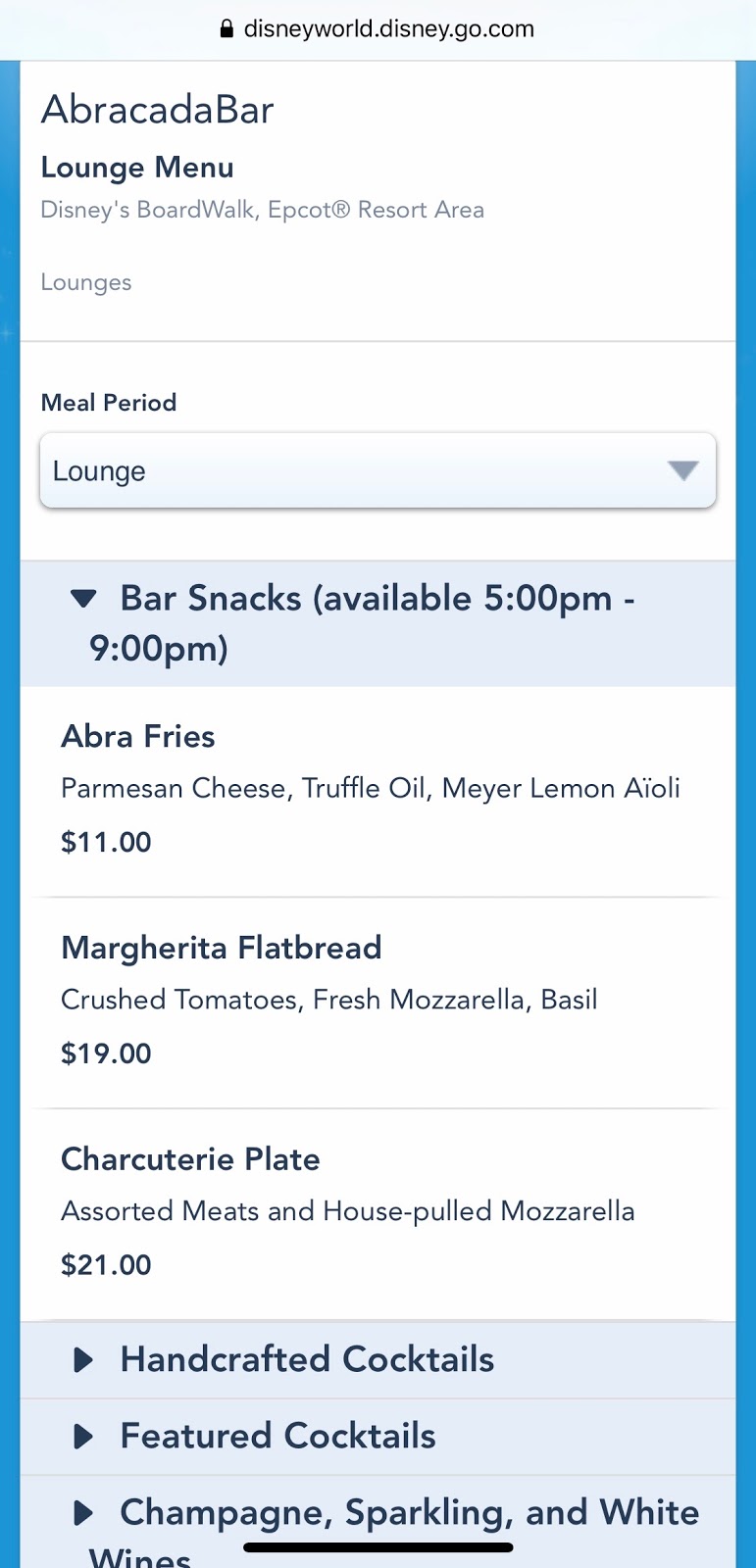The image displays a Disney World menu from the "AbracadaBar" located at Disney's Boardwalk in the Epcot Resort Area, accessible through the web address DisneyWorld.Disney.Go.com. The menu is prominently labeled with "A-B-R-A-C-A-D-A Bar" followed by "Avocado Bar". Below this heading is the "Lounge" menu section which specifies its location and details various lounge options. 

The menu lists the availability of bar snacks from 5 PM to 9 PM, beginning with:
- **Abra Fries**: A dish featuring Parmesan Cheese, Truffle Oil, and Meyer Lemon Aioli, priced at $11.
- **Margherita Flatbread**: A flatbread topped with Crushed Tomatoes, Fresh Mozzarella, and Basil, priced at $19.
- **Charcuterie Plate**: A selection of assorted meats paired with house-pulled mozzarella, priced at $21.

Additionally, there are three highlighted drop-down options:
1. Handcrafted Cocktails
2. Featured Cocktails
3. Champagne, Sparkling, and White Wines

These sections allow guests to explore a variety of beverage options to complement their lounge experience.